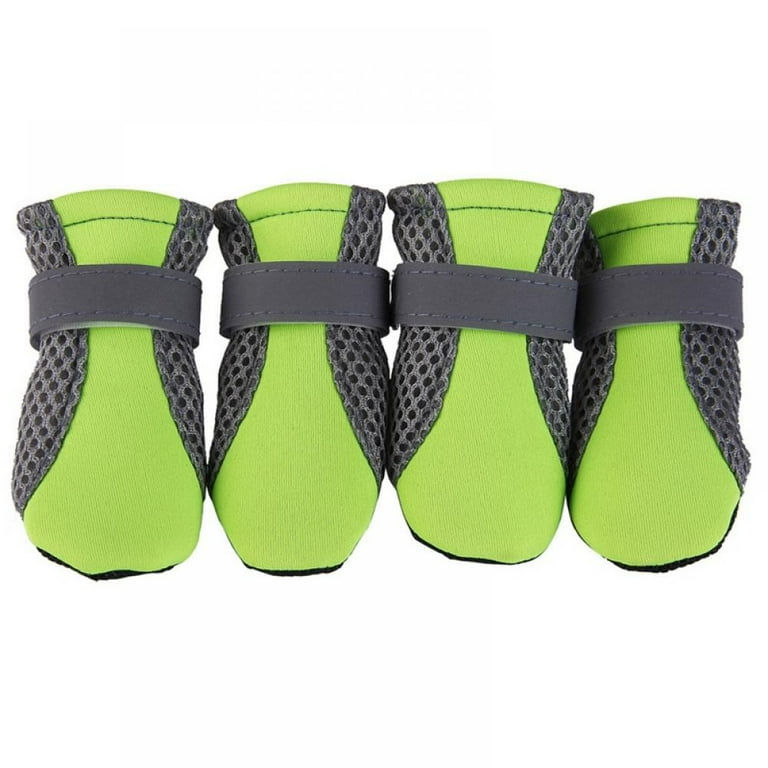The photograph showcases a close-up view of four identical dog boots arrayed in a straight line against a stark white backdrop. Each boot features a vibrant neon green front and is encased in a black mesh around the sides. A central black strap allows for adjustable tightness around the dog's paws. The underside of the boots appears to be made from a different black material, likely designed for durability and comfort, akin to a sandal, providing protection for an injured paw during its healing process. The boots are free of any visible letters or numbers and the entire scene is brightly lit, highlighting the detailed textures and colors of the boots clearly.